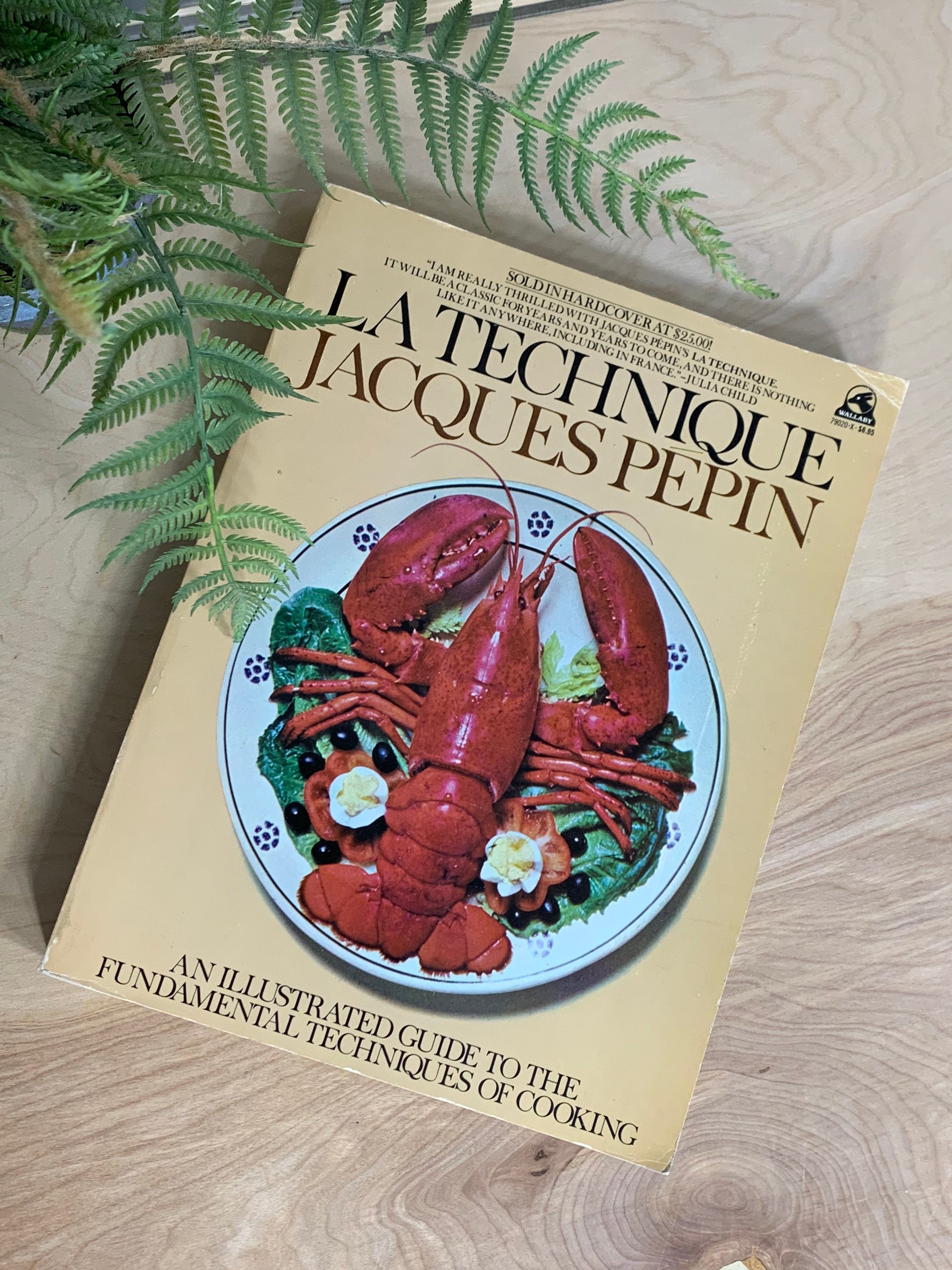The photo captures a diagonally placed book on a light brown wooden tabletop, featuring a strong, natural knot in the wood. At the top left corner of the image, there are ferns, which could be either real or artificial, enhanced by the presence of a potted plant beside the book. The book cover prominently displays a vibrant picture of a cooked red lobster resting on a bed of green lettuce, accompanied by eggs, black olives, tomatoes, and other garnishes. The title "La Technique Jacques Pepin" is clearly seen at the top of the cover, with the subtitle "An Illustrated Guide to the Fundamental Techniques of Cooking" written below the lobster image. The background of the book cover is a striking yellow, adding a warm and inviting contrast to the detailed culinary imagery. The book is priced at $25, and is noted to be a classic culinary guide, praised for its timeless techniques.